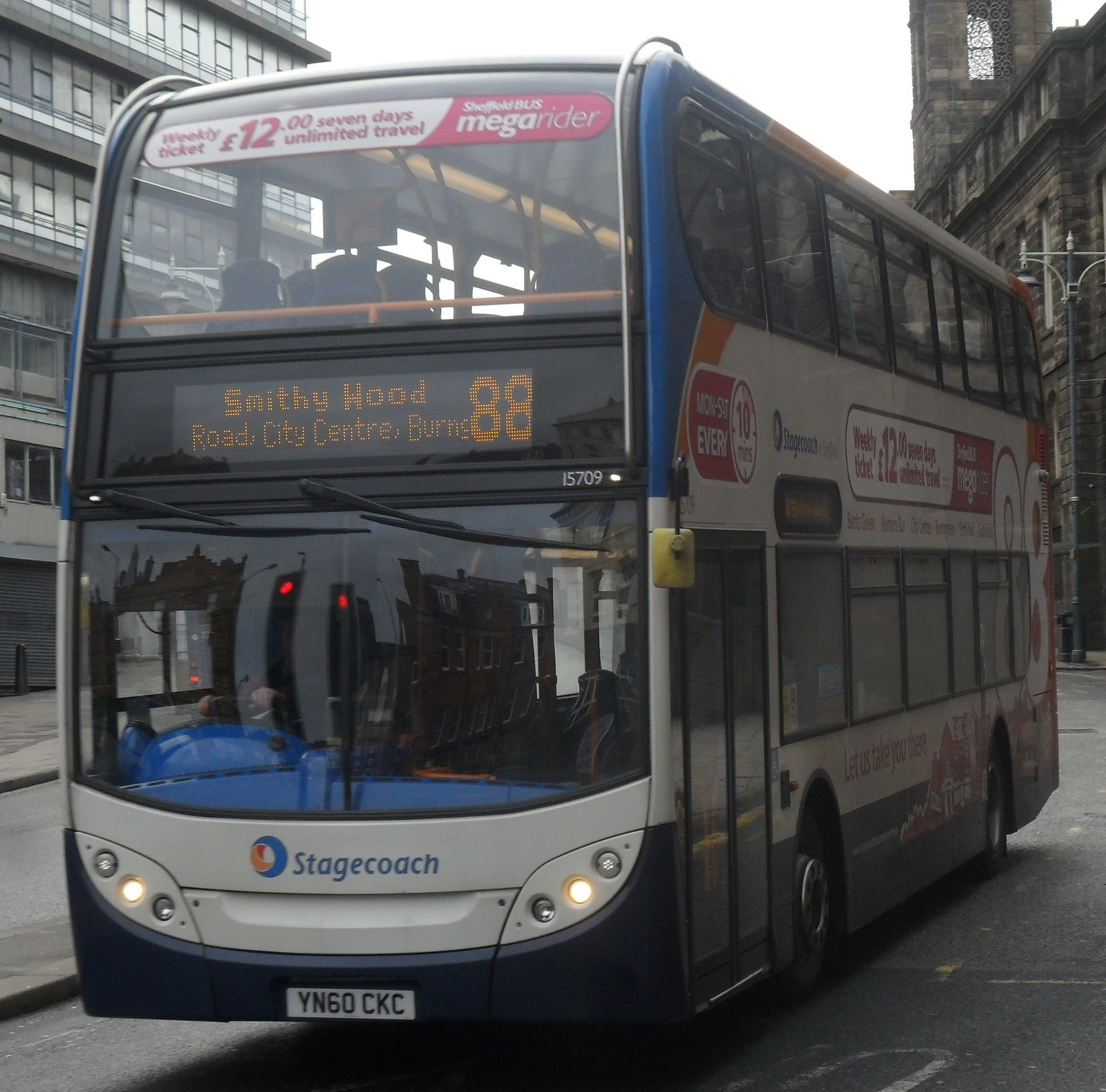A modern double-decker bus, predominantly gray with dark blue outlines, is pictured up-close facing left on a paved street. The bus, number 15709, prominently displays the "Stagecoach" logo at the front along with a blue, orange, and red circular emblem. Its large front windows and numerous side windows suggest a lack of passengers, save for the driver. Above the windshield, a digital sign reads "Smithywood Road, City Center, Burns 88," indicating its route number 88. The white license plate reads YN60CKC.

The bus features distinctive circular headlights that house different lights such as the high beams, running lights, and turn signals. The bus is adorned with various advertisements on its side in red and white lettering, offering promotions like "Weekly Ticket, €12, 7 days unlimited travel, Sheffield Bus MegaRider" and schedules reflecting frequent services. Similar signage is present on the right side of the bus, including a prominent "Let us take you there" slogan. The rear right bears a large number "88" with a red outline, reinforcing its route. 

The photo's backdrop includes multi-story buildings on either side, with a stark white sky above them, situating the bus in an urban environment.